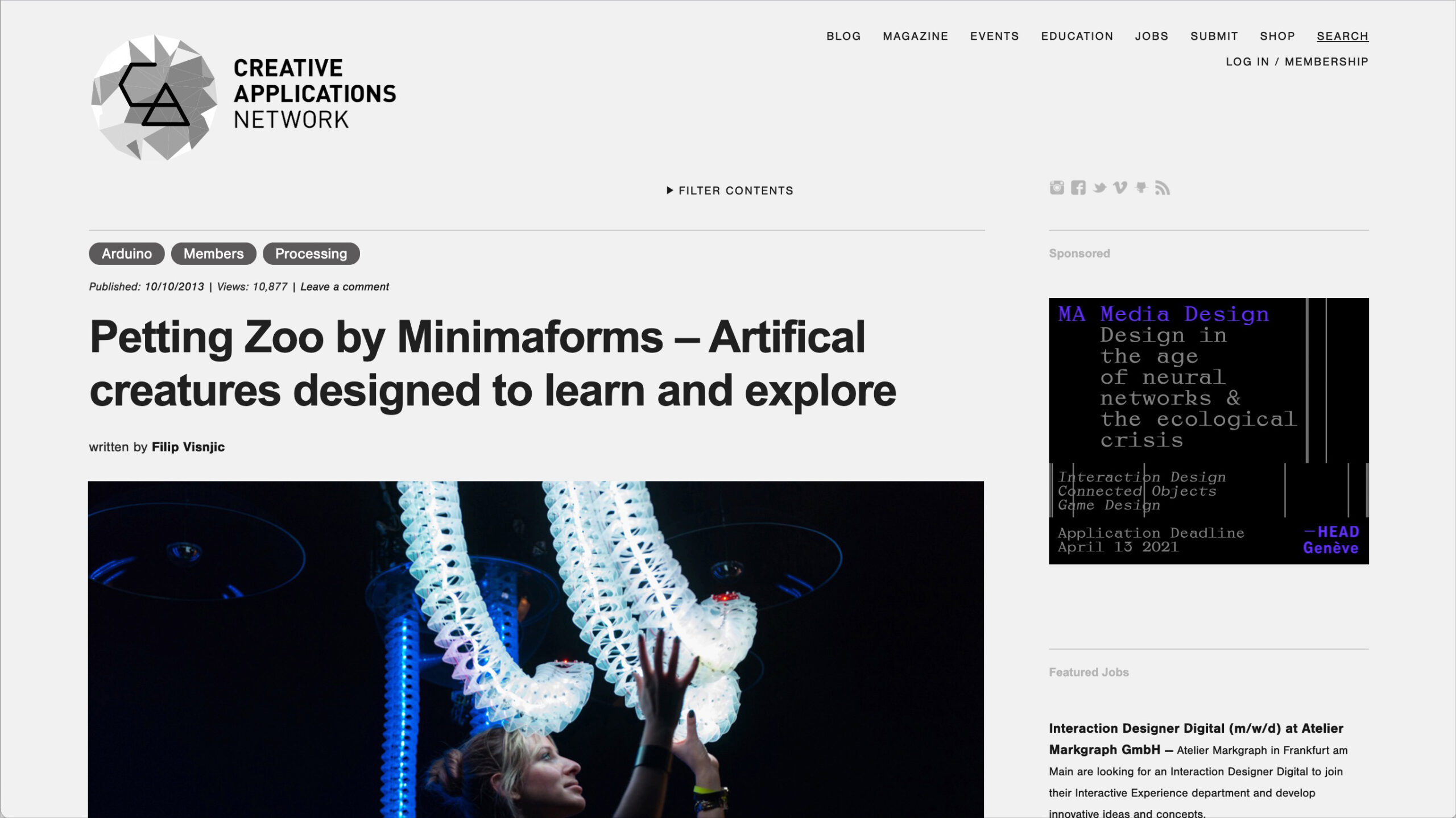The image portrays a detailed layout of a website in color, featuring a predominantly beige background. In the top left corner, the website is branded as "Creative Applications Network" with a logo adjacent to it resembling a diamond viewed from above, marked with the initials "CA" at the top. In the top right corner, several navigation tabs are visible, labeled Blog, Magazine, Events, Education, Jobs, Submit, Shop, and Search.

Scrolling further down the page reveals a featured article published on October 10, 2013, which has garnered 10,877 views. The article, available for comments, is authored by Filip Janjic and headlines as "Petting Zoo by Menema Forms: Artificial Creatures Designed to Learn and Explore." On the right sidebar of the webpage, there is sponsored content and featured job listings, including a position for an Interaction Designer in Digital.